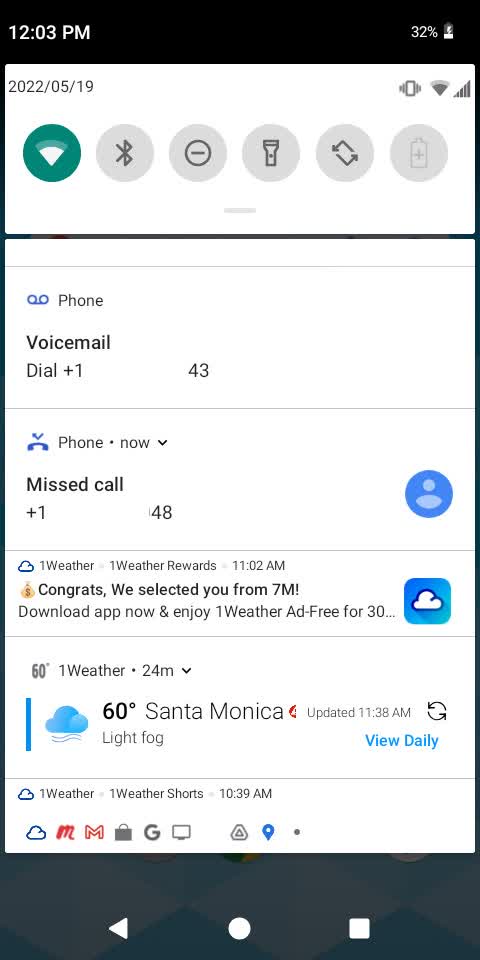The image appears to be a screenshot from an Android or Google phone, taken at 12:03 PM. The status bar at the top indicates that the battery is at 32% and currently charging. The background at the very top of the screen is black, transitioning to a white rectangular widget area below. This widget area includes buttons for Bluetooth, flashlight, a Do Not Disturb icon (a circle with a horizontal line through it), and Wi-Fi. The date displayed is May 19, 2022.

On the right side of this widget area, there is a faded-out battery icon. At the bottom of the screen, there is a section showing a voicemail notification with a prompt to dial a number, partially obscured for privacy, followed by a blank space and the sequence "43 pin." Just below this, there's a notification for a missed call from a partially redacted number, showing the number "+1 [redacted] 48." Accompanying this is a blue circle with a person icon. 

Finally, the weather app indicates it is 60°F in Santa Monica with light fog.